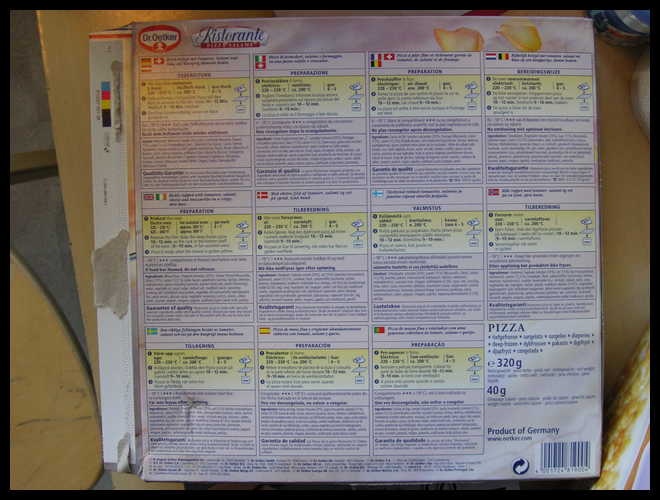The image depicts the back of a pizza box, which has been opened. The box is square and predominantly white. On the bottom right-hand side, the word "Pizza" is prominently displayed, followed by text that reads "320G" and "40G" underneath it. At the very bottom, it states "Product of Germany." In the top left-hand corner, there is a red logo with a white center, although the text within the logo is illegible. Next to the logo, the word "Restaurant" appears, written in blue. The main area of the box is covered with extensive text, divided into multiple squares—four across the top, four across the middle, and three across the bottom, but the text in these squares is too small to discern.